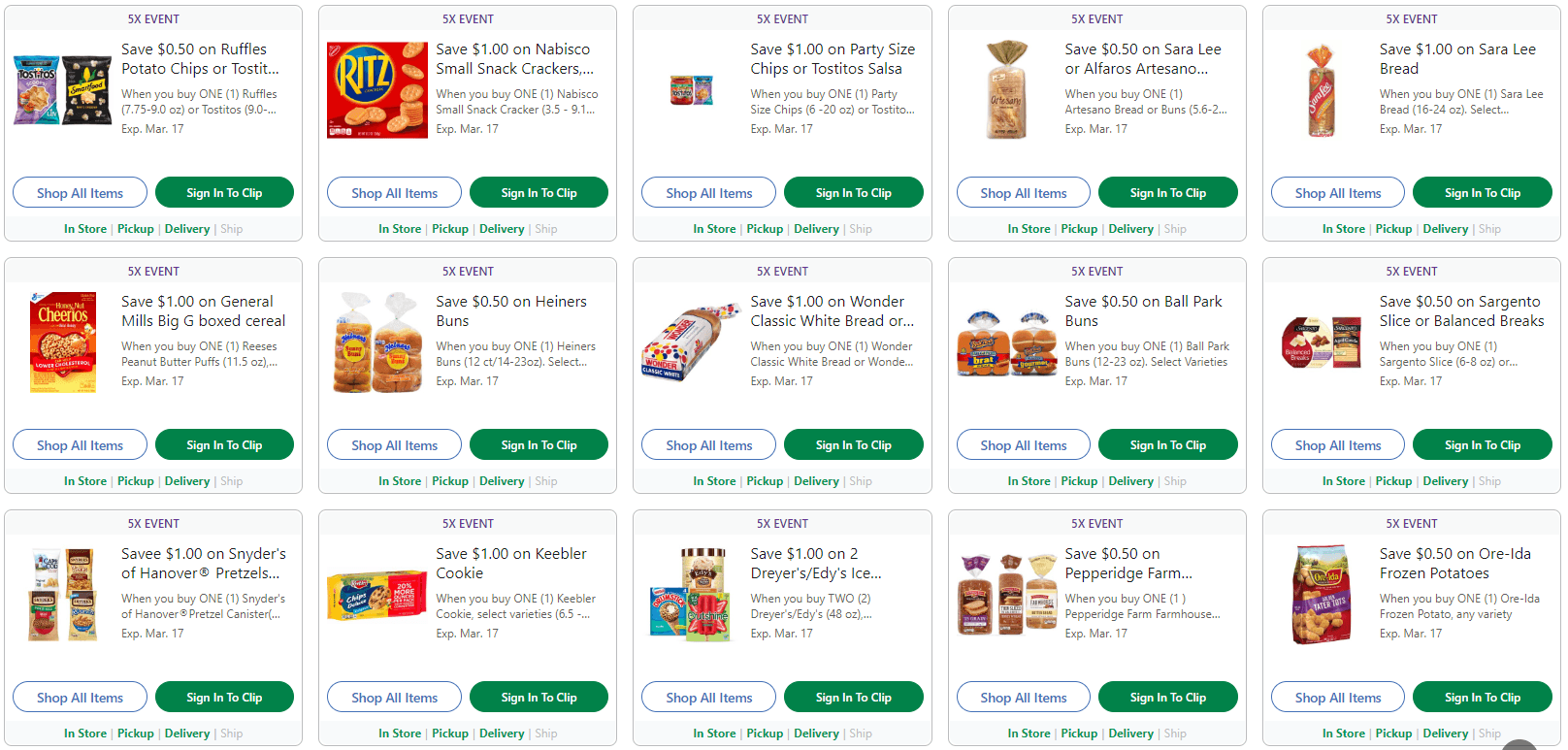A detailed screenshot of what appears to be an online shopping website, possibly Instacart, showcases a selection of grocery items. The interface features a clean white background with a grid displaying a total of 15 products arranged in five rows by three columns. Among the visible items are Ritz crackers and hotdog buns, each accompanied by a product photo, a product header, and a single line description. At the top of the grid, a prominent green button labeled “Shop All Items” stands out. The overall layout and design elements suggest a user-friendly platform tailored for convenient online grocery shopping.